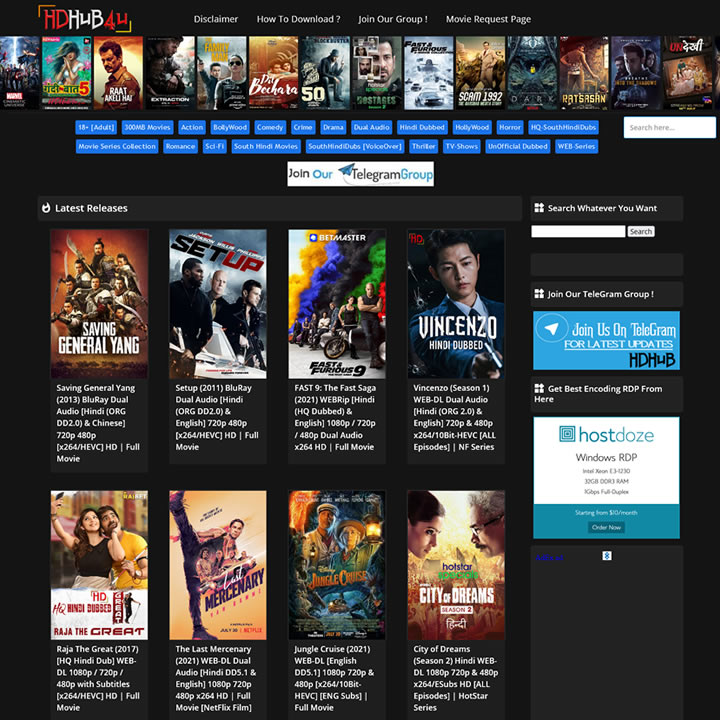In this small and somewhat cluttered presentation, the topmost section features a line of text in various bold colors and cases: "HD" in red uppercase, followed by "HUB" in white with a lowercase "u," and then "4U" in red with a lowercase "u." Below this header, there are 14 thumbnails of movie posters arranged in a single horizontal row. Each poster seems to be a snapshot of different films. Above these thumbnails, you can discern several navigation options including "Disclaimer," "How to Download," "Join Our Group," and "Movie Request Page."

Underneath the row of movie posters, the layout shows a segmented area where various categories are selectable. To the right side of this section, there's a search bar for easy navigation. Centered directly below is a prominent white bar with an invitation to "Join Our Telegram Group." Further down, there are two rows of movie thumbnails, four in each row, each accompanied by brief descriptions.

On the right-hand side, there are additional options to join the Telegram group and a section labeled "Hostos." The overall design seems geared towards user interaction, providing multiple points of access and information dissemination.